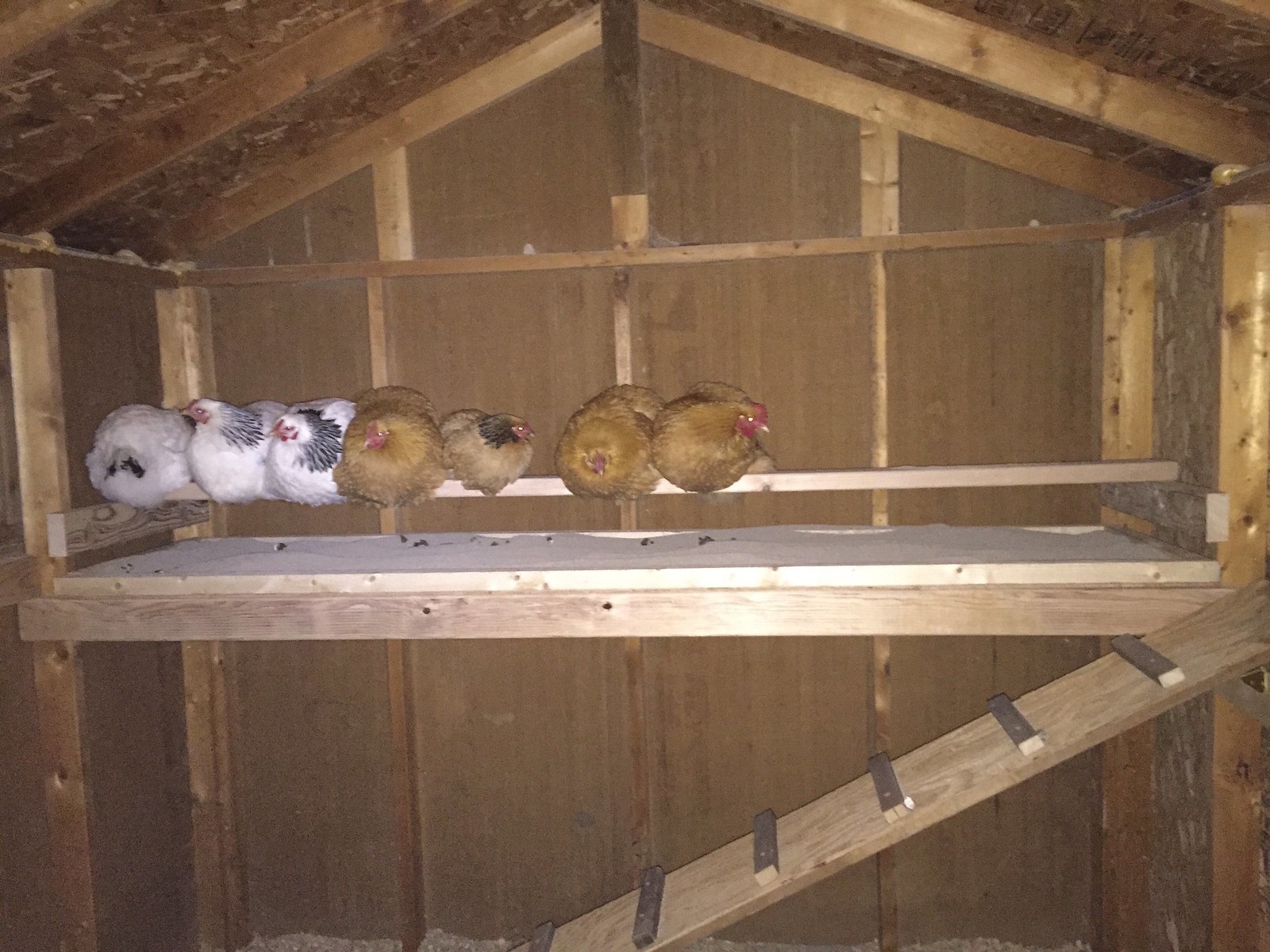The image depicts a detailed view inside a meticulously crafted wooden chicken coop with a tilted roof. The coop has been designed to allow a clear view inside, possibly with the front removed. Inside, a wooden perch runs horizontally, occupying the middle section, while a small platform beneath offers additional support. A sloped ramp featuring regularly spaced steps extends from the bottom middle to the right edge of the image, providing the chickens easy access to the perch.

Resting on the perch are seven live chickens, all facing the camera. They are aligned closely together, showcasing a mix of vibrant plumage. Starting from the left, there are three white and black chickens followed by a brown chicken, a distinct brown and black chicken, and finally, two more brown chickens. The interior of the coop is notably clean, and the chickens appear comfortable and well-cared for. Their feet are concealed as they sit cozily side by side, enjoying their serene environment.